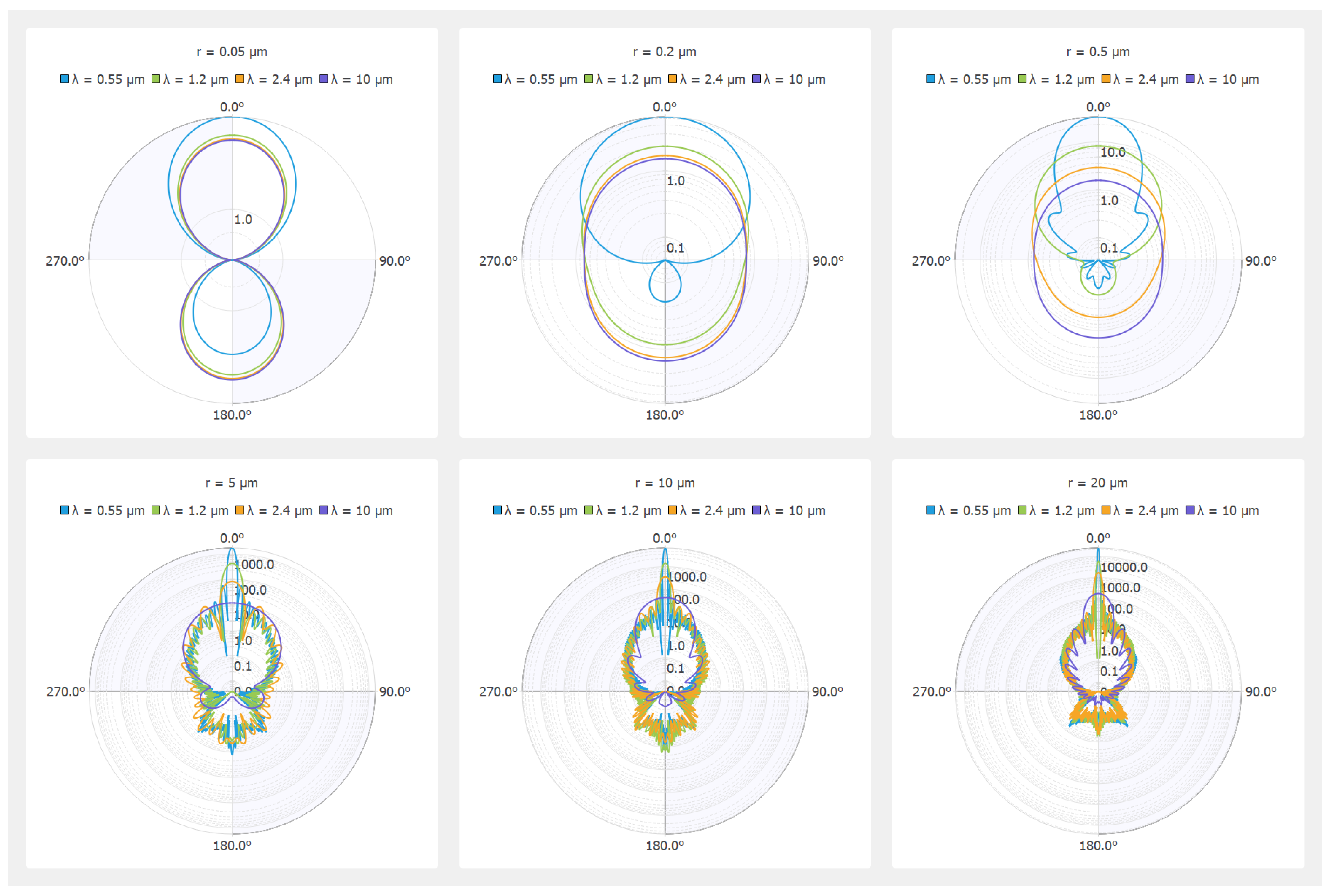This image features a series of six scientific diagrams, arranged in two rows of three diagrams each. Each diagram contains a primary gray circle, marked with degree notations: 0° at the top, 90° on the right, 180° at the bottom, and 270° on the left. Within these primary circles, variously colored secondary circles are depicted in different configurations. Each diagram includes a legend at the top that explains the color coding and their corresponding measurements in micrometers. For example, in the upper left diagram, the legends indicate that the blue circle represents a measurement of 0.55 micrometers and the green circle signifies a measurement of 1.2 micrometers. These specific measurements and color codes are consistent across all six diagrams. However, there is no explicit labeling or contextual information available to specify the exact nature or subject of these diagrams.